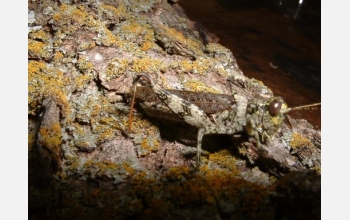The image is a close-up photograph, likely taken to showcase camouflage, featuring a small, possibly grasshopper-like insect. The insect appears to be climbing on a lichen-covered rock. The rock itself displays various shades of brown, tan, and beige, interspersed with seafoam green and golden yellow lichens. The insect blends almost seamlessly into this mottled background, making it difficult to distinguish. Its body has a mottled pattern of gray and brown, helping it to almost disappear against the rocks. The insect has oval black eyes, antennae, and what appears to be a webbed foot for gripping the rock. The photograph has dark areas at the bottom and top right, and the background is dark brown, suggesting that the image was possibly taken at night with some illumination. There also appears to be another similar creature partially visible in the background, hinting at another camouflaged presence.